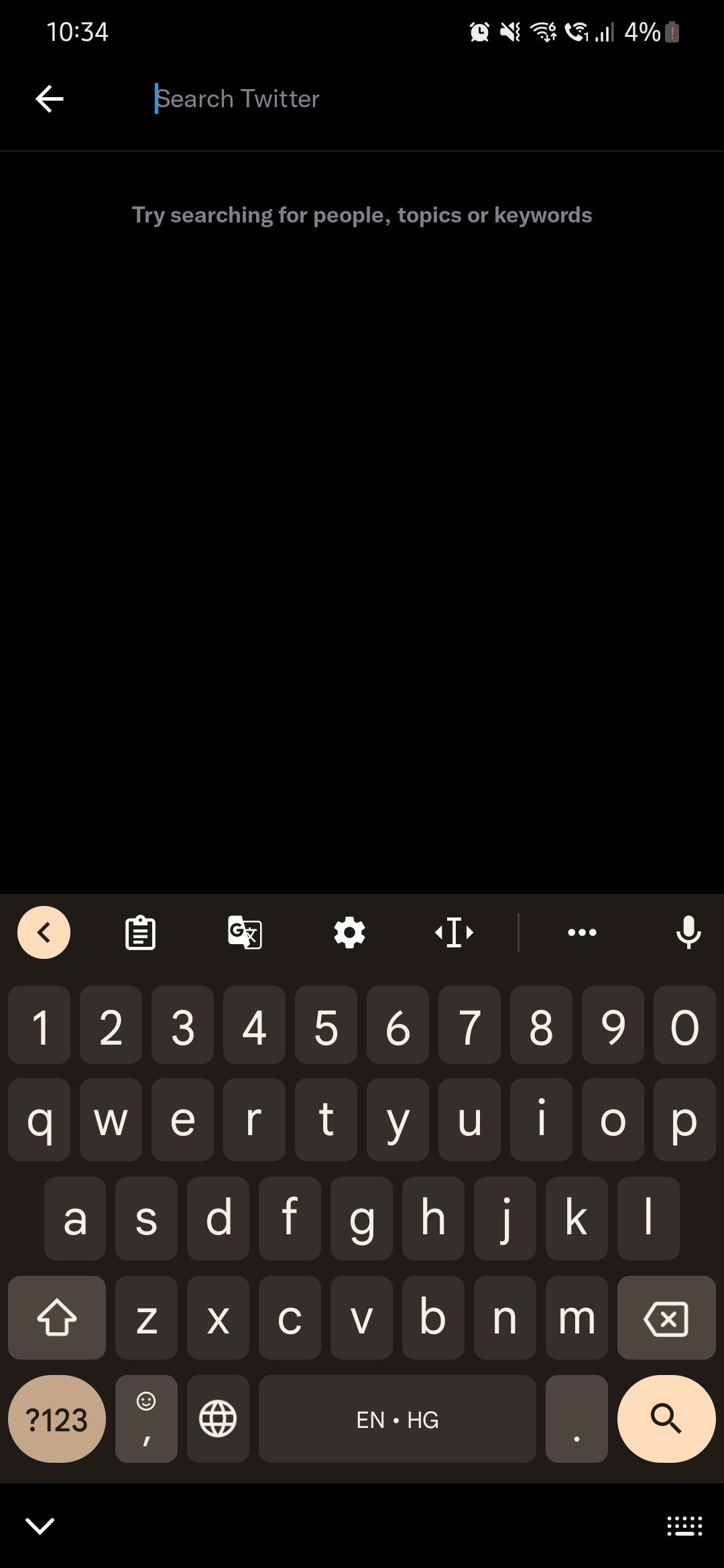Screenshot of the "dark mode" Twitter interface, with a black background. At the top left corner, the time is displayed as 10:34. On the same row, at the top right corner, there are six icons: an alarm clock, a vibrate icon, a cellular data icon, a call icon with one missed call, a Wi-Fi signal icon, and a battery icon showing 4% remaining. Below the icons, there is a search bar with the text "Search Twitter" and a blue cursor, accompanied by a white arrow pointing left. Below the search bar, there is a prompt saying, "Try searching for people, topics, or keywords." The rest of the page is blank.

At the bottom of the screen, there is a grey QWERTY keyboard with an additional number line above the letters. On the bottom left of the keyboard, there is an oval button labeled "123" and a question mark. The space bar is centered, and on the bottom right, there is a magnifying glass icon within a circle. The number button and the search button both have a white background, contrasting with the grey keys.